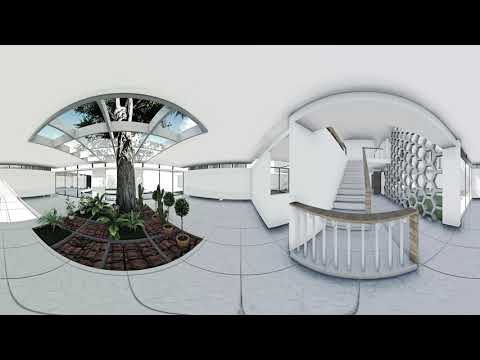The image presents a fascinating view, possibly utilizing a double fisheye lens, that captures two distinct yet connected scenes within a modern building's foyer. On the right side of the image, a sleek white staircase ascends, bordered by banisters with wood accents. Adjacent to the stairs, a striking honeycomb-patterned wall divider serves as a stylish barrier, providing a semi-transparent view through its intricate design. The ceiling above this area is enclosed and white.

Shifting the focus to the left side, an impressive atrium is showcased. Here, a tree extends majestically through an open section of the roof, allowing for an interplay of indoor and outdoor elements. This open-roof design complements the smaller plants and meticulously trimmed topiary that adorn the ground. The garden-like space is juxtaposed against the pristine white walls and gray tiled flooring, blending natural and architectural beauty. Beyond this indoor garden, glass walls and windows hint at exterior doors, suggesting an entrance into the building.

The entirety of the foyer, with its dual displays of modern architectural features and integrated natural elements, creates an inviting and contemporary ambiance, punctuated by the unique layout and detailed design elements.